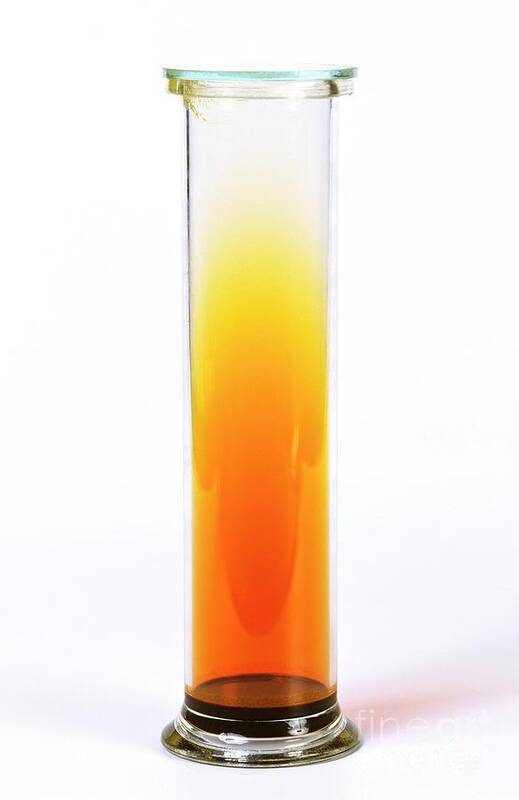The photograph showcases a slender, clear test tube-like object, resembling both a vial and a modern glass vase. The base appears to be a combination of black and silver. A small amount of dark liquid is present at the cylindrical base. Rising from this base, the tube features a dynamic, amorphous pattern in varying shades of orange and yellow, ascending approximately three-fourths of the way up the tube. The coloration on the glass surface seems more painted than liquid, forming a thicker oval-shaped area in the middle. The entire object is set against a pristine white background, which includes subtle shadow details. Additionally, a faint, whitish watermark reading "fine art" is discernible, blending almost seamlessly with the white surface. The test tube or vial does not have a lid, and the clear glass reflects its surroundings subtly.